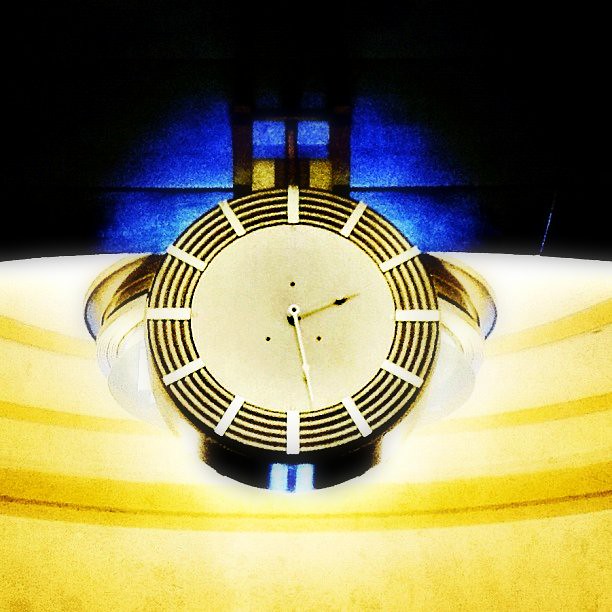The image depicts a highly stylized clock mounted on a yellow wall with a complex, striking design. The clock has a broad black base, adorned with gold semi-circular shapes extending to the left and right, somewhat resembling the insides of canoes. The clock face features a yellow background with concentric black circular stripes extending along its edges, adding depth and visual intrigue. The numbers are represented by simple gold rectangular bars, extending horizontally in place of traditional numerals. The clock hands are extremely thin and gold-colored, showing the time as approximately 2:27. At the bottom of the clock, there's a blue light at the base, which appears glossy and dome-shaped. The yellow wall, upon closer inspection, seems to be a layer with another blue surface behind it, possibly mimicking steps or adding a layered architectural element to the background. The overall impression is of a computer-generated image rather than a photograph, given the precise and highly stylized elements.